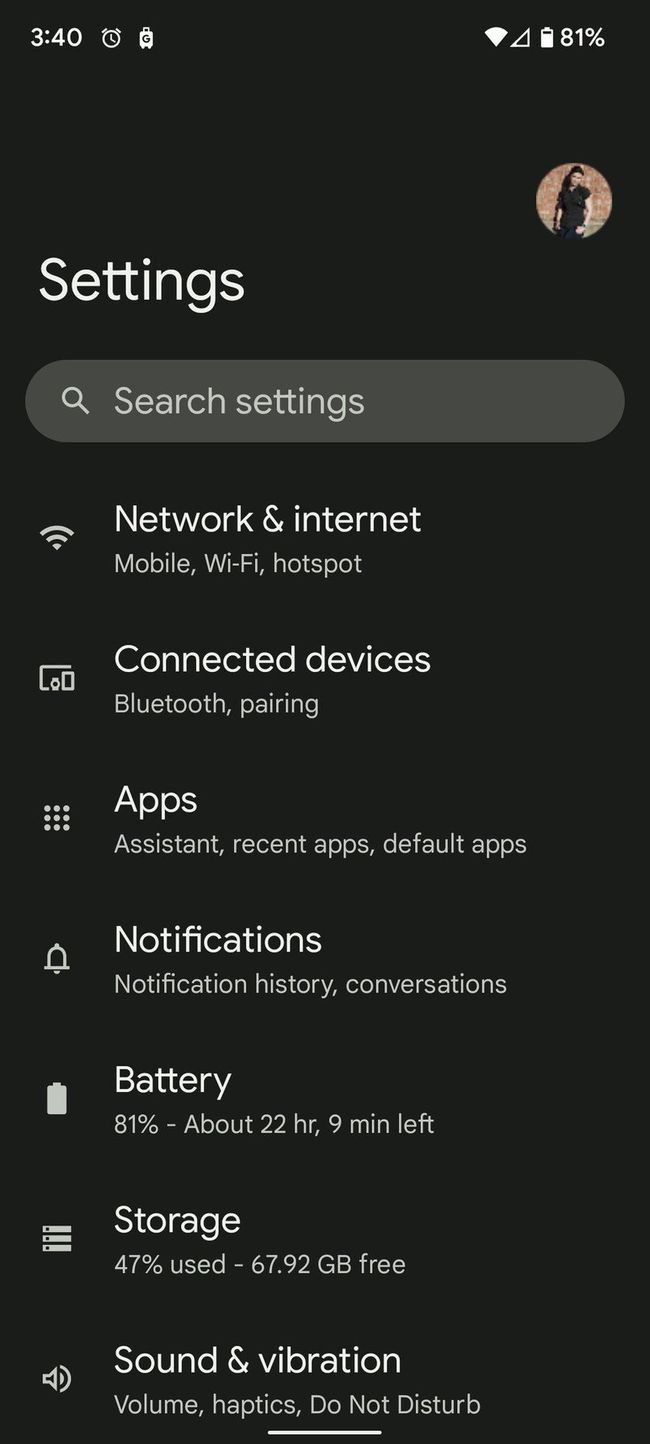This screenshot captures the settings menu of a smartphone, evident from the header text "Settings" displayed prominently in large white letters on a black background, suggesting the device is in night mode. At the top-left of the screen, the time reads 3:40, while the top-right indicates an 81% battery level. In the same top-right corner, there’s a small profile picture of the device's owner, showing two individuals—a man and a woman—posing outdoors against a brown background, both wearing black shirts.

The settings menu features a search bar labeled "Search settings," allowing users to efficiently find specific options without navigating through multiple tabs. Below the search bar, several main categories are listed sequentially: "Network & internet" for managing mobile data, Wi-Fi, and hotspot connections; "Connected devices" for managing Bluetooth and paired devices; "Apps & notifications"; "Battery"; "Storage"; and "Sound & vibration." Each category provides access to specific settings related to its function, ensuring users can customize their phone’s configuration with ease.